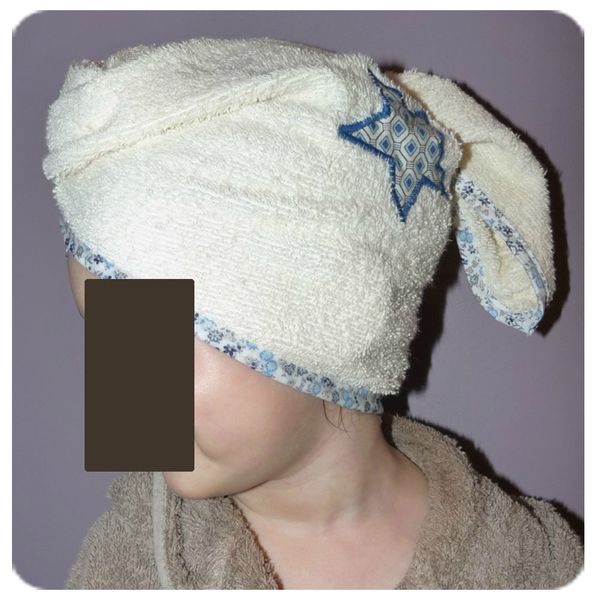In this photograph, a woman is seen standing against a solid purple wall, her shadow prominently cast upon it. Her face is obscured by a small black rectangular bar, masking her eyes, nose, and mouth. Her hair is wrapped in a white towel adorned with a blue star on top, and a few damp strands are visible at the bottom of the wrap. The towel features a blue floral fringe pattern. She is wearing a brown fuzzy robe or towel around her neck and shoulders. The image, which has curved corners, depicts her from just below the neck up, evoking the sense that she might be fresh out of the shower. The clear and detailed depiction of the head wrap and its design suggests the possibility that this photograph could be intended for advertising the head wrap itself.